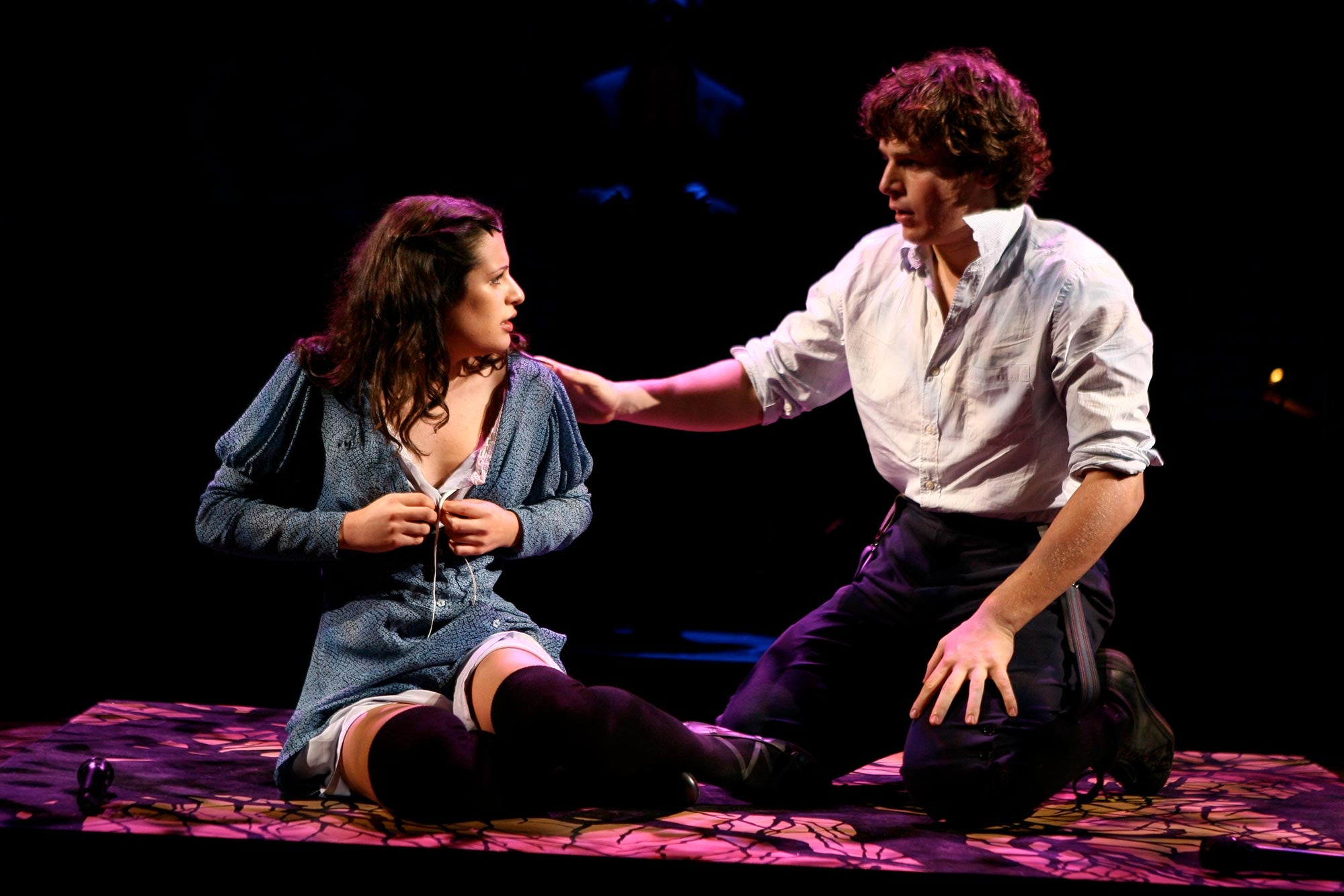This is a color photograph capturing an intense and dramatic moment between two actors on stage, likely from a theater production. The scene is bathed in diffused pink, purple, and blue lighting, casting a stained glass-like pattern on the ground beneath them. The woman, seated on the floor to the left, has long dark brown hair reaching her armpits. She appears concerned as she buttons up her blue dress, which features a V-neck bodice. Her legs, bent at the knees, are off to the side, and she's wearing black tights. The man, kneeling to her right, has voluminous, curly brown hair. He wears a white button-up shirt with the sleeves rolled up to his elbows, black pants, and brown boots. With his right hand gently placed on her left shoulder and his left hand resting on his knee, he looks at her with a mixture of worry and intensity. The background is dark, accentuated by blue lighting, adding to the emotional weight of the scene.